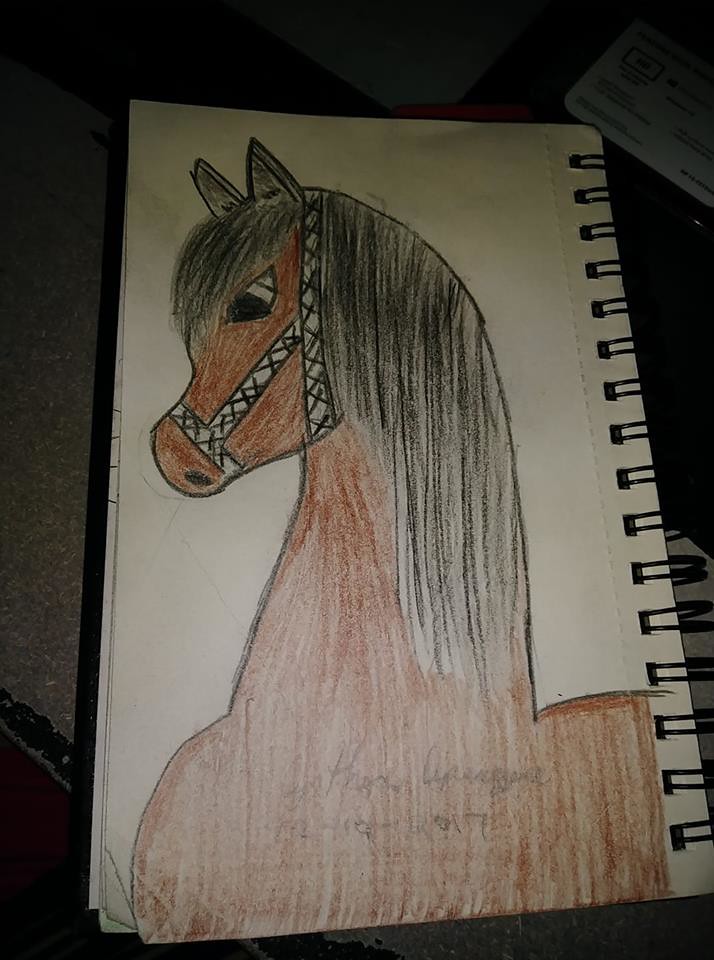The image showcases a detailed drawing of a horse, sketched with colored pencils on a white sheet of paper from a spiral-bound sketchbook. The artist has rendered the side profile of the horse, capturing its head, neck, and the upper part of its body. The horse's body and face are predominantly brown, colored with vertical lines, while its mane and ears are black. The mane flows straight down from its head with a noticeable section on its forehead. The horse appears to be wearing a black bridle with a criss-cross pattern around its muzzle and nose, and its eyes are depicted in black and white, gazing downward to the left. The neck of the horse is illustrated as large and muscular. The background remains blank white, and at the bottom of the drawing, there seems to be a barely discernible name and date, written in grayish pencil.